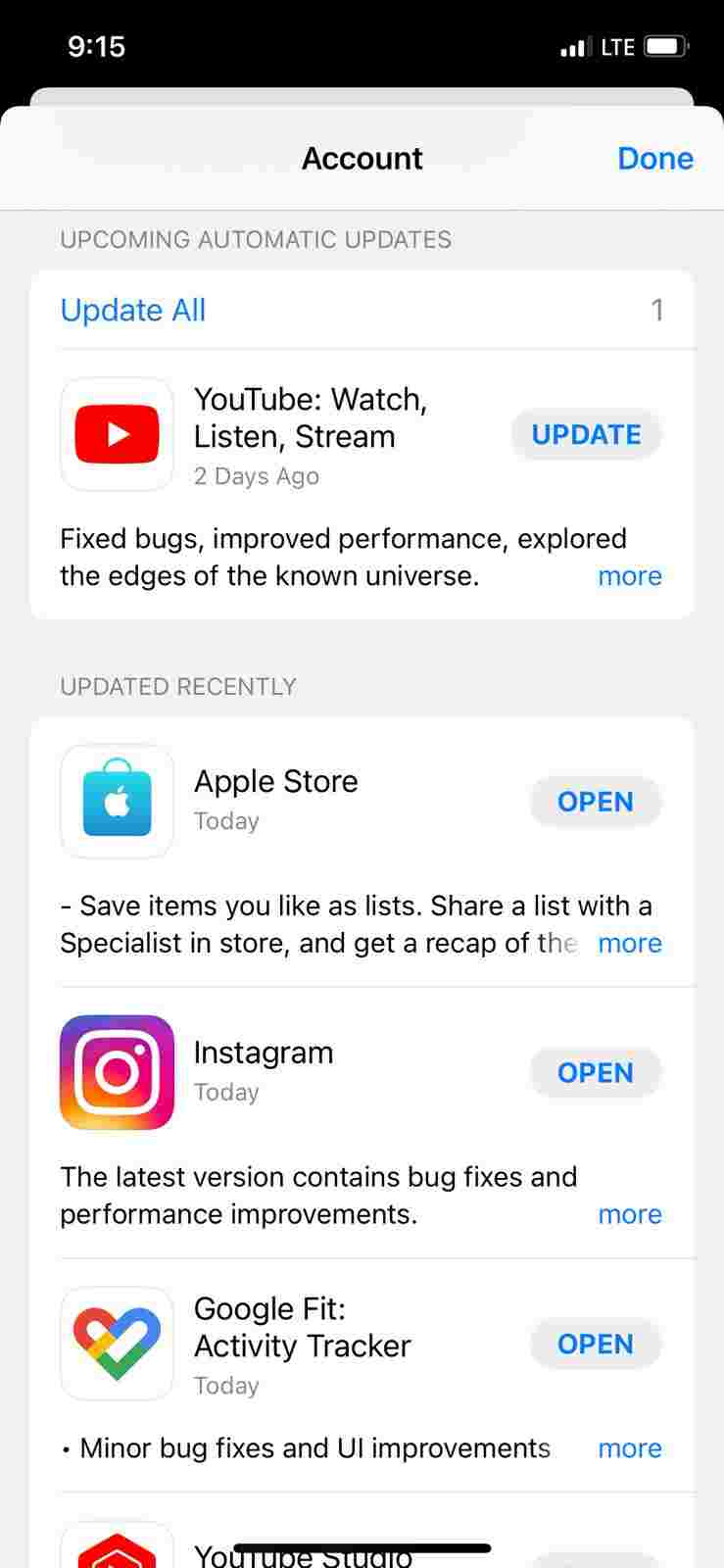The screenshot depicts the screen of a phone, identifiable by the top bar displaying common phone interface elements. On the left side of this bar, the time reads 9:15. The right side includes symbols indicating LTE data connection and battery status.

The main content of the screenshot is an iPhone display showing an App Store page with a prominent white tab labeled "Account" at the center. To the right of this tab is a blue "Done" button. Directly below, a heading states "Upcoming Automatic Updates," followed by a list of apps requiring updates. The first app listed is YouTube, showcasing its logo on the left and the app name on the right, alongside details about its last open time and the improvements included in the update.

Further down, another section labeled "Updated Recently" lists several apps including Apple Store, Instagram, Google Fit, and YouTube Studio. Each of these apps features an "Open" button next to their names on the right, except for the YouTube app at the top which has an "Update" button instead. This section also provides information on when these apps were last used, which in most cases is "Today," and details about the most recent updates.